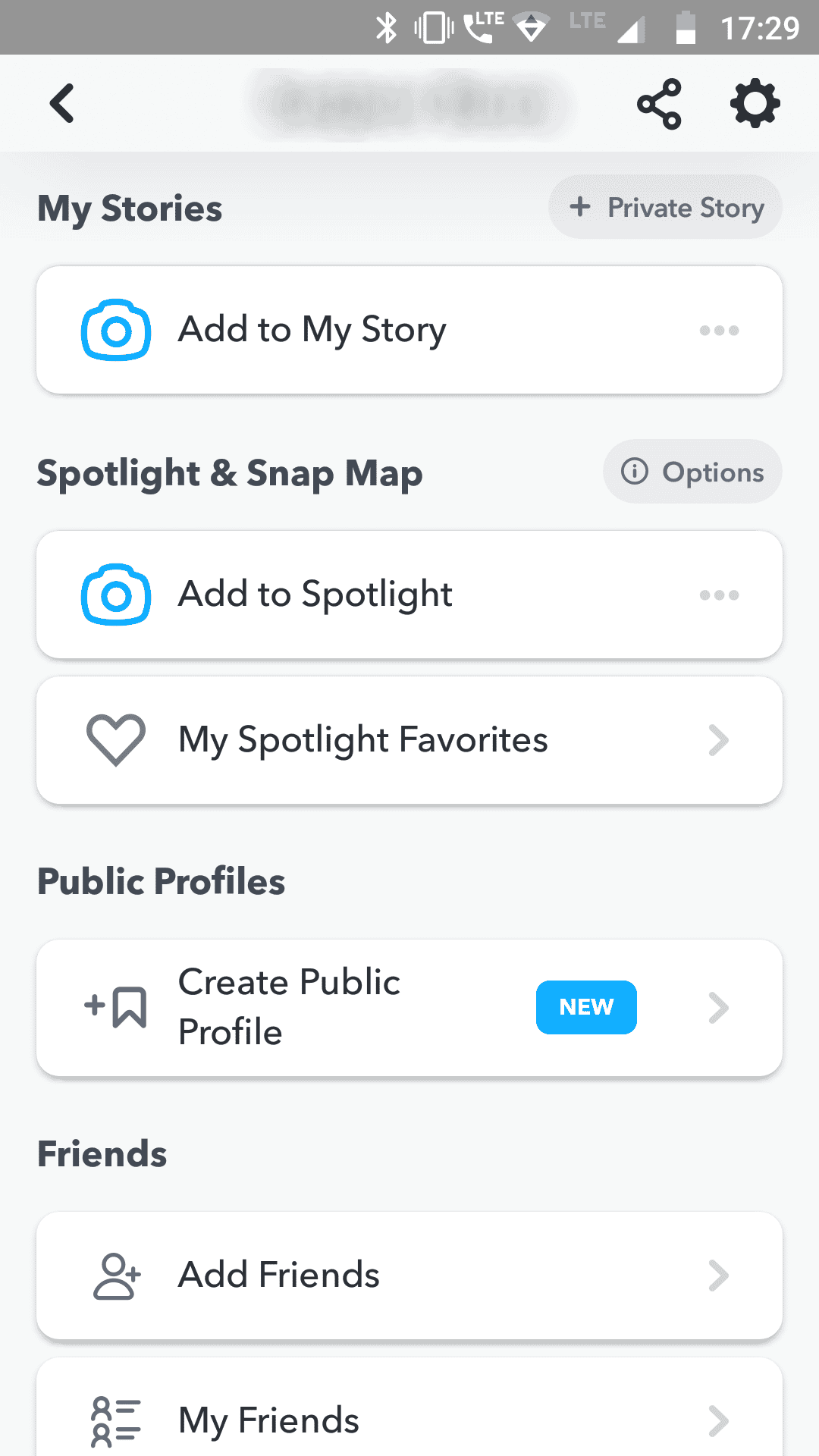This is a detailed image of a smartphone screen, likely an Android device, captured in a wide and long format. At the top, the status bar displays several system icons: the Bluetooth icon, a screen rotation icon, a general phone icon, and a Wi-Fi signal indicator showing about three-quarters strength. Beside these, there's an LTE indicator, nearly full signal strength bars, and a half-full battery icon. The time “17:29” is displayed next to these icons.

Below this, on the left-hand side, there's a left-pointing arrow, indicating a back function. On the right-hand side, there are share and settings icons. 

The main body of the screen is divided into four sections. The first section titled "My Stories" includes a button for creating a private story on the right, displayed as a plus sign inside an oval button. "My Story" is highlighted within a white rectangular area accompanied by a picture icon.

The second section is labeled “Spotlight and Snap Map”. This section is split into two parts: one for adding content to Spotlight and another labeled “My Spotlight Favorites”.

The third section titled “Public Profiles” features an option to create a public profile, noted as “New”.

The fourth and final section, labeled “Friends”, contains options to “Add Friends” and “My Friends”, each with appropriate icons corresponding to their functionality.